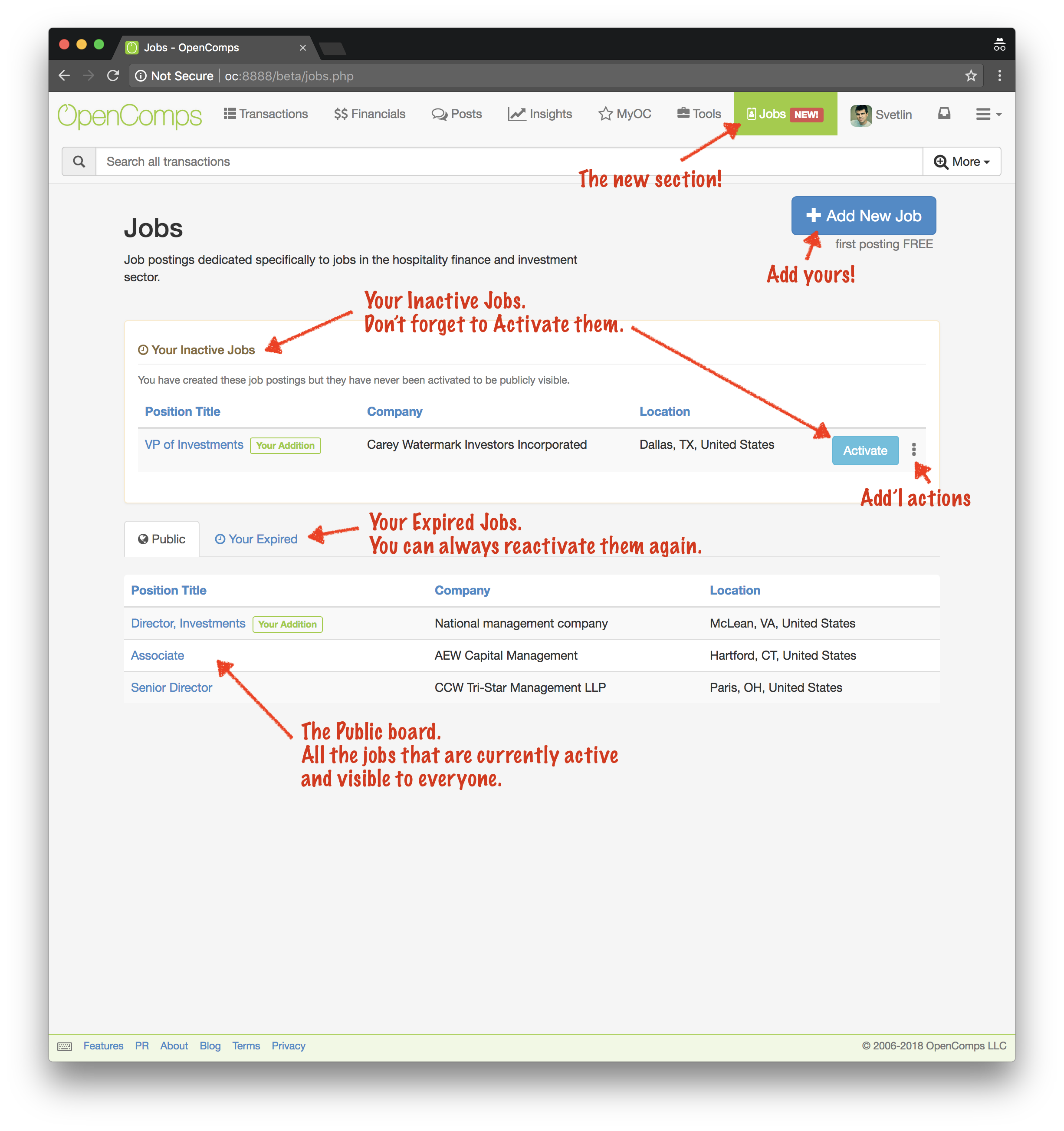This image is a screenshot of the OpenComps website, displayed in a Chrome browser with a green icon on the tab. The website interface is clean, featuring a white background with gray font for the menu items. The top menu highlights options for Transactions, Franchise, Posts, Insights, MyOC, Tools, Jobs, and displays the name of the logged-in user.

Directly below the menu, there is a search tool for querying transaction data. A notable feature within the screenshot is a red arrow and text indicating a new "Jobs" section, pointing towards the relevant tab. In the upper right corner of the jobs section, red text marks an "Add yours" option, inviting users to post new job listings.

The "Jobs" section is currently selected in the screenshot. This section focuses on job postings related to the hospitality franchise and investment industry. Errors are indicated by arrows pointing to both inactive job listings with a prompt to activate them. Explicit instructions suggest users not to forget to activate their inactive postings, with actionable options adjacent to this reminder.

Below the activation prompt, there's a section for reviewing expired job listings, which can be reactivated if necessary. Finally, the job listings are organized in a table format with columns for Position Title, Company, and Location. The public job board displays all active and publicly visible job postings.